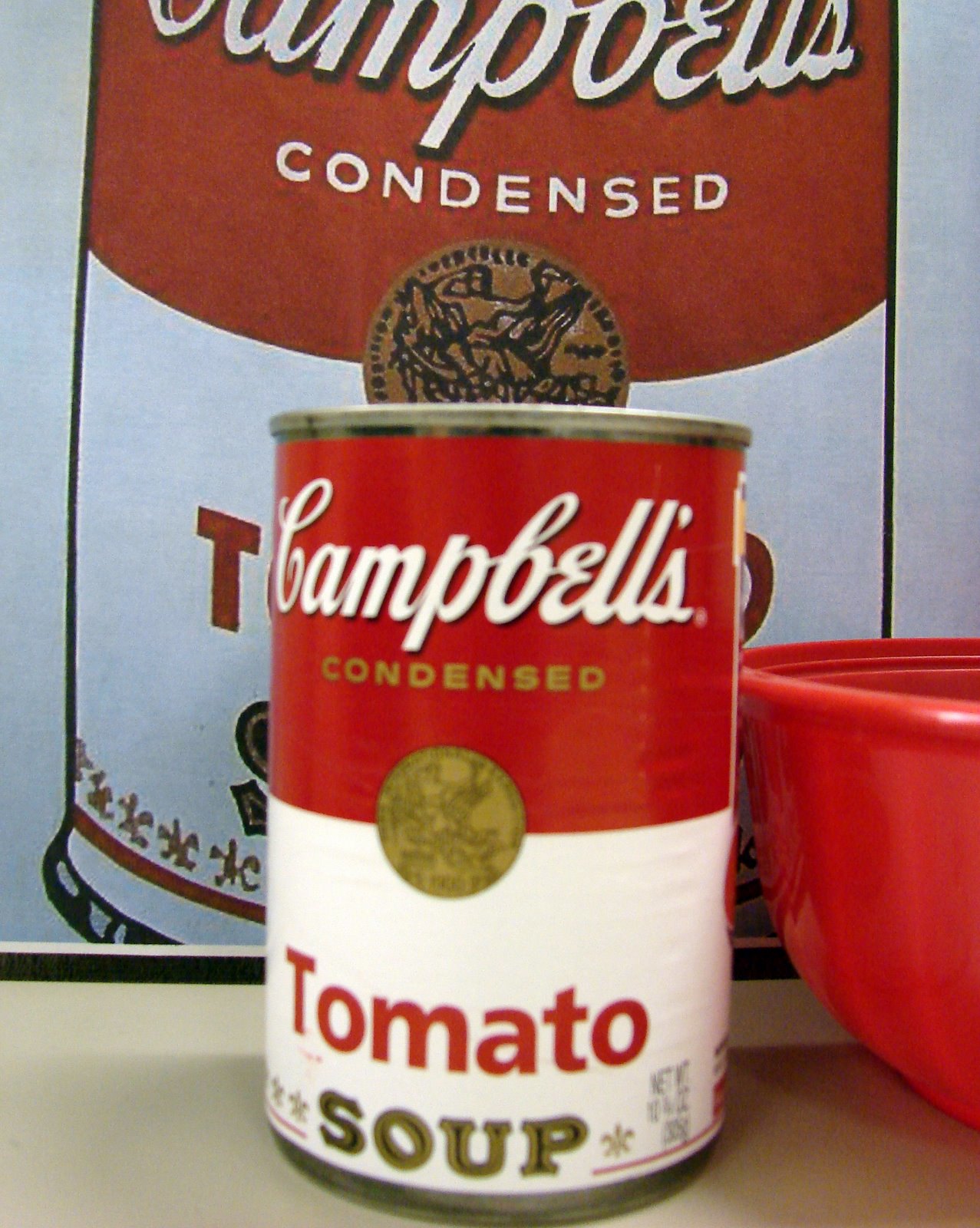The image showcases a classic can of Campbell's condensed tomato soup, prominently displayed on a white countertop. The can features its iconic design: a silver base with a red and white label, "Campbell's" emblazoned in white, a golden medallion in the center, and "Tomato Soup" written below. To the right of the can, a portion of a red plastic bowl is visible. In the background, a white piece of paper stands upright, displaying a hand-drawn illustration of a Campbell's soup can. The drawing replicates the can's details with markers, including the red top, white "Campbell's" logo outlined in black, and "condensed" written below. Additional features on the golden medallion, such as a person saluting, are also depicted, along with intricate details at the bottom of the can.